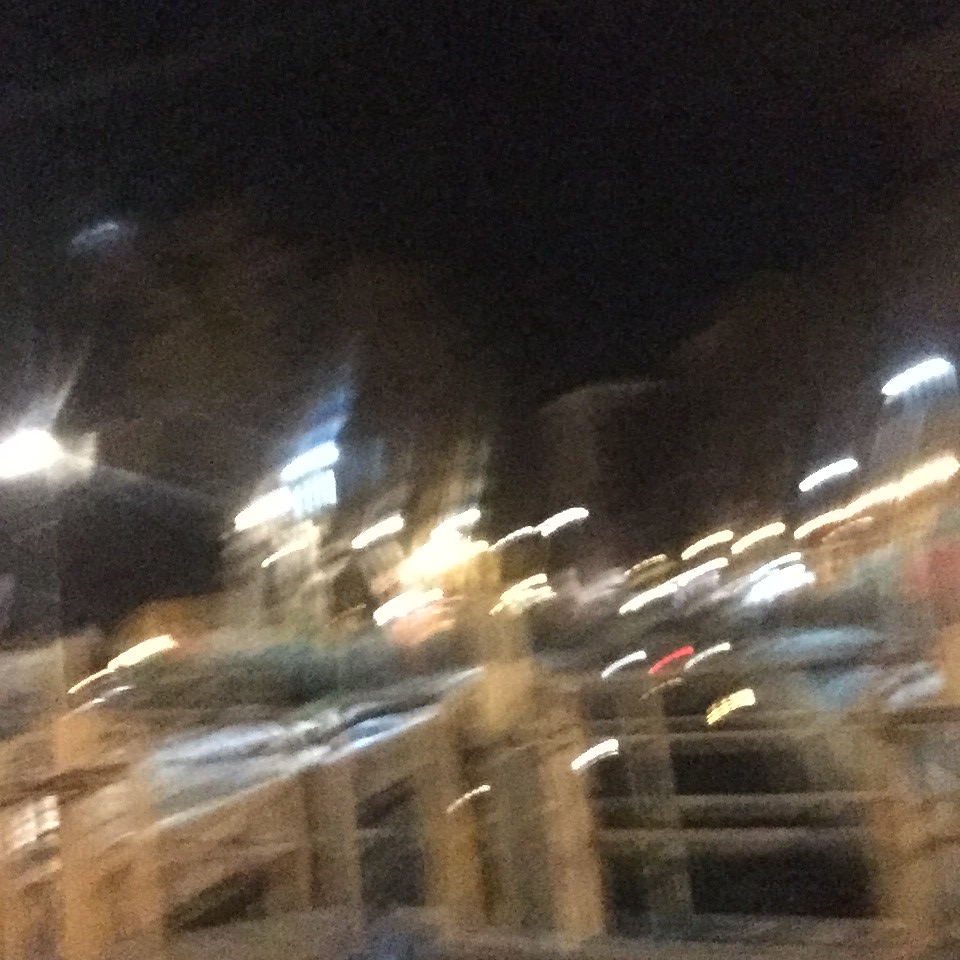A blurry photograph taken likely in a bustling downtown area. In the background, indistinct buildings with black rooftops are visible, adorned with horizontal, white lights that appear distorted due to the blur. The foreground showcases a broad sidewalk or walkway adjacent to a parking lot filled with parked cars, reinforcing the sense of an urban environment. The ambient lighting and the presence of multiple vehicles suggest a lively, active locale despite the lack of clear detail.